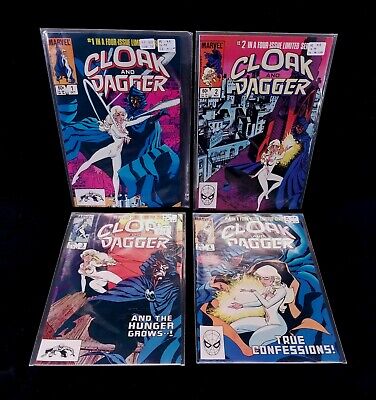The image displays a set of four Cloak and Dagger comic books prominently featuring covers with a heroine dressed in a white bodysuit and fairies or women in body suits. These comics are titled "Cloak & Dagger," "True Confessions," and "The Hunger Grows." The vivid colors of pinks, blues, purples, whites, and blacks dominate the covers, which also have Spider-Man stickers on the bottom left-hand corners, indicating their Marvel Comics origin. Two of the comics are lying flat on the ground, while the other two are standing upright against a black background. They are possibly collector's editions, as they are wrapped in plastic, hinting that this might be an advertisement for selling these comic books on an e-commerce platform such as eBay.